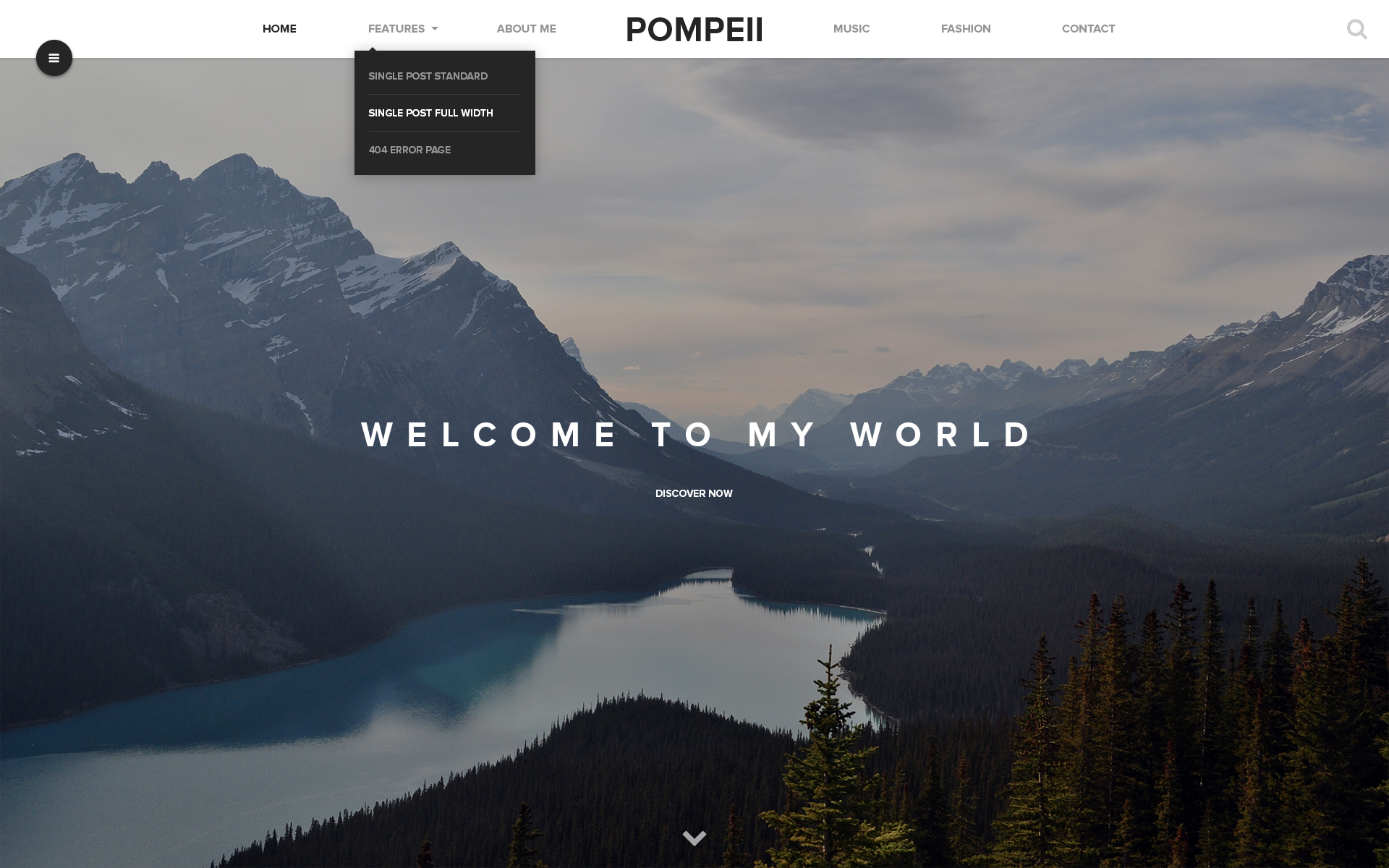Sure! Here's a cleaned-up and detailed caption based on the provided description:

---

"This webpage, titled 'Pompeii,' features a top navigation bar with tabs labeled (from left to right) Home, Features (with a drop-down arrow), About Me, Music, Fashion, and Contact, along with a search bar. On the far left, there is a hamburger menu icon and a black circle. The page's background displays a breathtaking valley scene with mountainous terrain beneath a cloudy sky. Snow-capped peaks, brown in hue, frame the landscape, enhancing its majestic beauty. A serene lake and a dense forest are also visible, complementing the natural splendor. Overlaid in white text are the words 'Welcome to my world' and an invitation to 'Discover Now.' At the bottom of the page, a down arrow prompts visitors to scroll further. The Features tab's drop-down menu includes options for Single Post Standard, Single Post Full Width, and Full 404 Error Page. The website is named 'Pompeii' and is spelled P-O-M-P-I-E-I-I."

---

This version organizes the information logically and adds descriptive details to enhance the visual presentation.